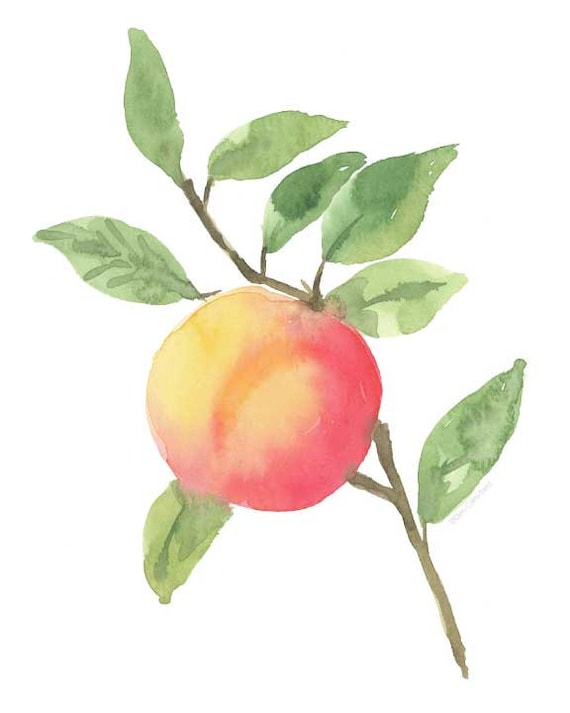This detailed watercolor painting depicts a single, slender branch rendered in greenish-brown tones, devoid of any background or frame. The branch, extending diagonally from the bottom right to the top left corner of the canvas, supports eight green leaves, which lack intricate definition and are symmetrically placed along both sides. At the heart of this composition is a fruit, ambiguously suggesting either an apple or a peach, nestled at the branch's center. The fruit showcases a beautiful gradient, transitioning from a rich red on one side to a mellow yellow on the other, with subtle hints of orange. The entire artwork is set against a simple, unembellished white background, enhancing the focus on the central elements of the branch and fruit. The painting exudes a serene simplicity, free from any textual distraction.